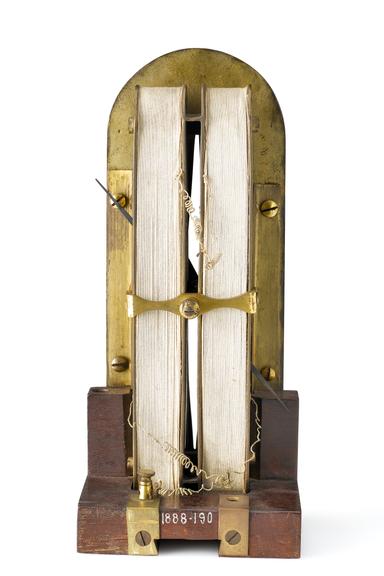The vertically aligned rectangular image depicts a vintage object set against a plain white background. Centered at the bottom, there is an aged-looking block of wood in a reddish-brown hue. This wooden base is flanked by two gold-colored metal brackets, each with a visible screw at the front edge. Between these brackets, the inscription "1888-190" is printed in white. Rising from this base, the central portion of the object resembles two standing books, viewed from the page side, held together by a horizontal gold bracket with a nail at its center. The bracket seems to allow the books to slide out or open like an accordion. Surrounding the upper part of these book-like elements is a gold metal frame that arches gracefully with four nails, two on each side. This mix of materials and intricate design gives the object a timeless and mysterious quality.